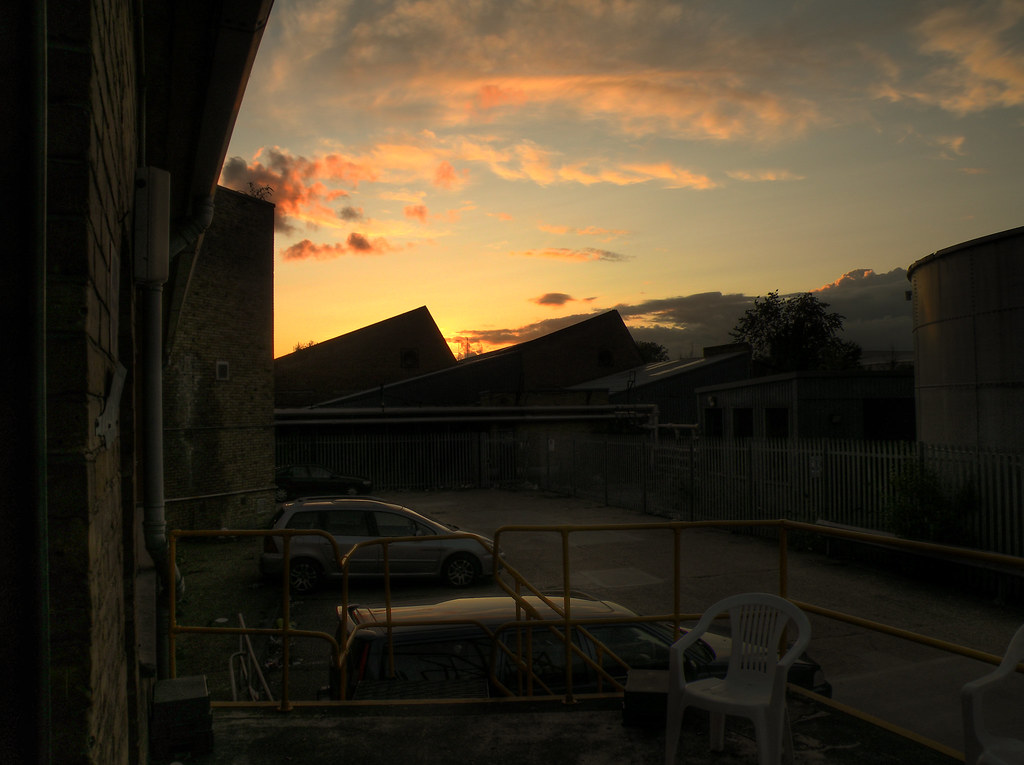This rectangular horizontal photograph captures the back of a workplace or a motel at dusk. The scene features a terrace with yellow metal or wire railings along its edges and a small white plastic lawn chair with a rounded back positioned in one corner. The surface of the terrace allows visibility through the beams and spaces. On the ground below, three SUVs or minivans are spaced out in a parking lot, all facing outward with their noses out. A wooden fence encloses the lot, and beyond it, there are other structures, including buildings that appear to be apartments. The side of the main building in the image reveals a bit of brickwork and a protruding pipe. Trees dot the background, interspersed with more buildings. The sky occupies the upper third of the photograph, displaying a light blue hue transitioning into golden coppery clouds, reflecting the setting sun. The sunset, casting a golden-yellow glow, almost completely vanishes behind the silhouetted rooftops and a distant mountain, creating a serene yet striking backdrop.